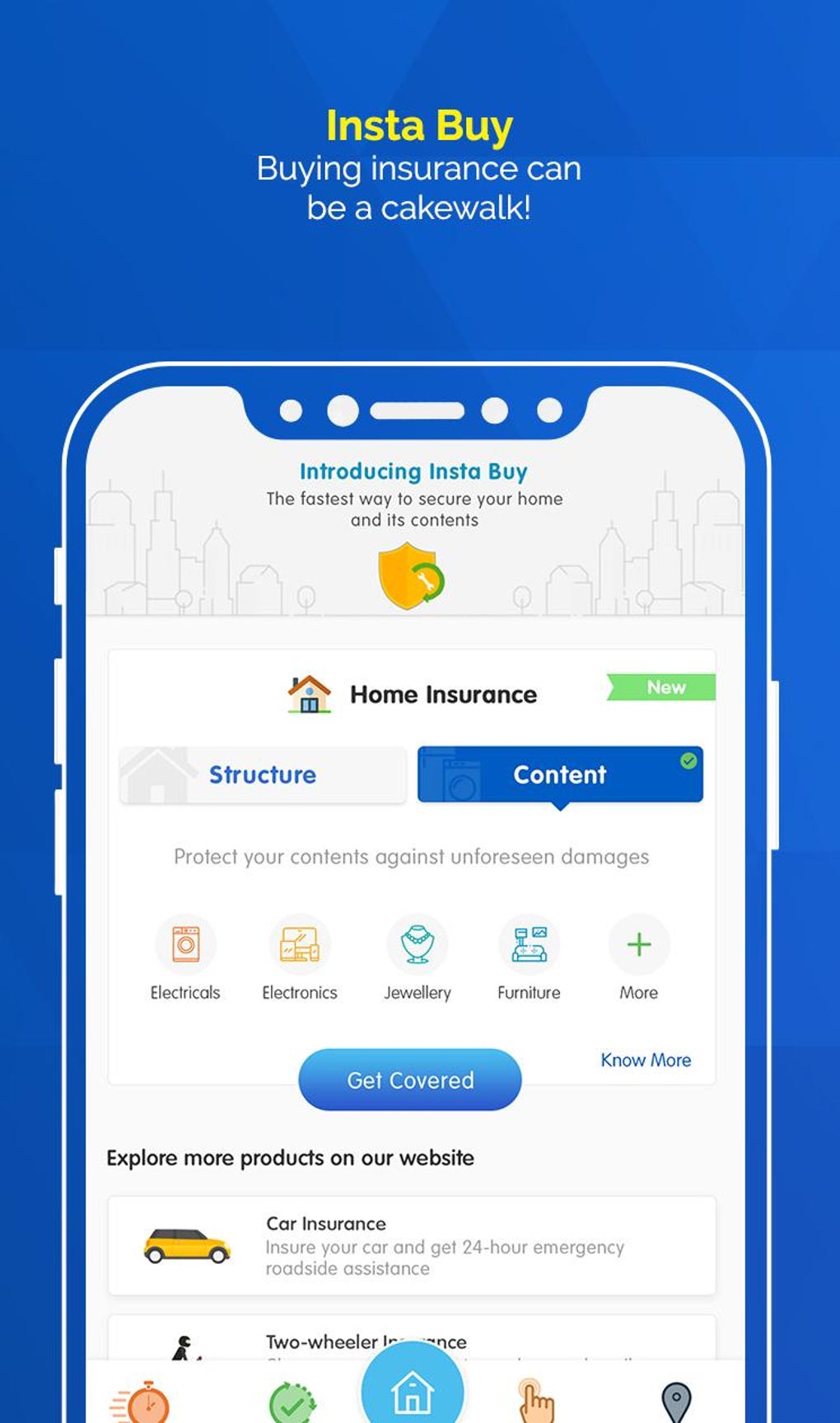**Image Caption: Detailed Advertisement for Home and Vehicle Insurance**

The image features a vibrant and visually organized advertisement emphasizing home and vehicle insurance. Dominated by a harmonious mix of blue, yellow, and green elements, it highlights various aspects and benefits of the insurance service.

In the upper section, set against a blue rectangle, the text “Buying insurance can be a cakewalk" is displayed in white, encouraging potential customers. Alongside this, the phrase “Introducing InstaBuy” is highlighted in blue text. Below this, a yellow badge with the label “Home Insurance” catches the eye, underscoring the primary focus. Accompanied by the tagline, “The fastest way to secure your home and its contents," it aims to convey ease and efficiency in the insurance process.

Towards the bottom, a green rectangle marked with the word “New” in white signifies a fresh and innovative approach to structure and content insurance, emphasizing the inclusion of both property and its contents. A gray rectangle specifies the "structure" component, indicating coverage for structural damages. Additionally, another blue rectangle concentrates on the "content" component, assuring protection against unforeseen damages to items like electronics, jewelry, furniture, and more.

Adjacent to this, a blue oval contains the directive “Get Covered” in white letters, reinforcing the call to action. Another blue oval further encourages exploration with the phrase “Explore More Products on Our Website."

In the bottom right corner, an illustration of a yellow car is paired with details about car insurance, including benefits like “insure your car and get 24-hour emergency roadside assistance.” Further information is provided in a blue circle mentioning coverage for two-wheelers, alongside an image of a house framed in white to symbolize home insurance offerings.

This comprehensive and vibrant presentation underscores the diverse insurance products available, highlighting user-friendly services and urgent assistance to potential customers.